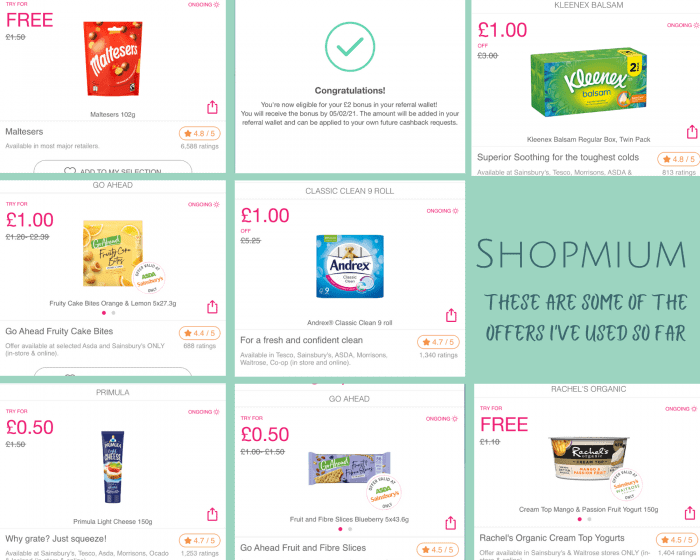In this screenshot of a sales and e-commerce site, we see a grid layout reminiscent of a tic-tac-toe design, featuring three rows and three columns demarcated by green lines. Each cell contains different items or messages, except for a couple of empty boxes. Here's a detailed breakdown:

### Top Row:
1. **Mattersters** - Features a red bag of snacks with a price listed (though the exact type isn't specified).
2. **Congratulations Message** - This cell congratulates the user on becoming eligible for a £2 bonus in their referral wallet.
3. **Clinics** - Displays a product related to clinics, priced at £1.

### Middle Row:
4. **Fruity Cake Bites** - Listed at £1, though the brand is unclear.
5. **Lemon Product** - Another item priced at £1, specifics not provided.
6. **Shop Him** - The box right in the middle of the row is empty but labeled "Shop Men, Shop Him."

### Bottom Row:
7. **50 Cent Item** - Contains an item priced at 50 cents.
8. **50 Cent Item** - Another item priced at 50 cents.
9. **Free Item** - This cell is blurred but displays an item listed as 'free.'

Each box includes small photos along with the price and brief information about each product, aiding quick decision-making for potential buyers.